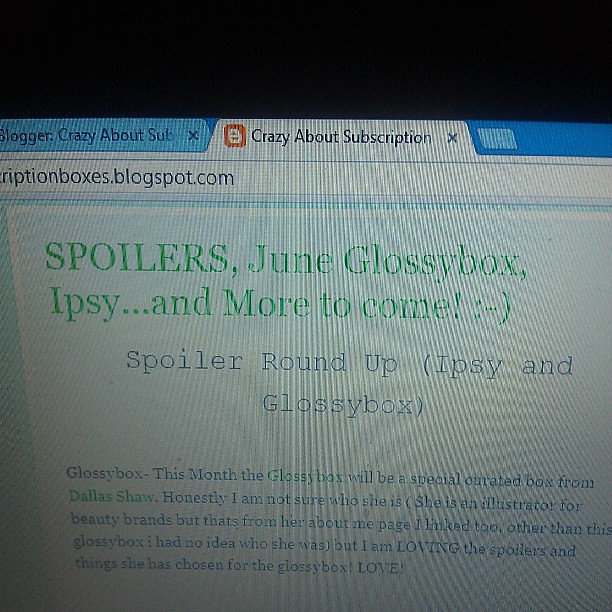This is a color photograph of a computer screen displaying a web page from the address subscriptionboxes.blogspot.com. The browser shows three tabs at the top: on the upper left, a blue tab with black text reading "Blogger Crazy About Sub"; in the middle, a white tab that says "Crazy About Subscription"; and on the right, a blank light blue tab. At the top of the web page itself, there is a section with green text on a white background that reads "Spoilers, June, Glossy Box, Ipsy, dot dot dot, and more to come :)". Below this, in larger blue text, it says "Spoiler Roundup: Ipsy and Glossy Box". A paragraph of smaller blue text follows, detailing that "Glossy Box this month will be specially curated by Dallas Shaw, an illustrator for beauty brands." The paragraph mentions the author's lack of familiarity with Dallas Shaw but expresses excitement about the chosen spoilers for the Glossy Box.